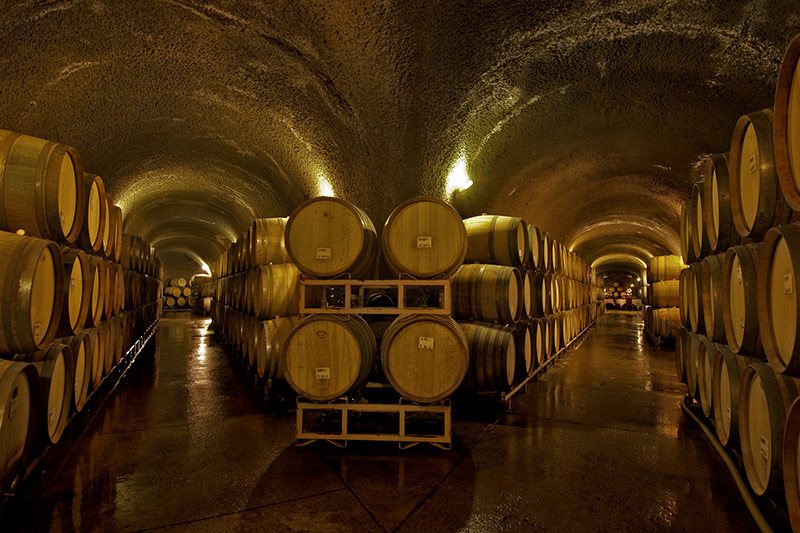The photograph depicts an underground winery cellar at a junction where a primary hallway branches into two separate tunnels, each lined with stacked wooden barrels. The tunnels feature stone, arched ceilings that rise just above the tops of the barrels, creating a cave-like ambiance. The barrels, positioned three high on either side and topped with brown labels, are arranged on beams or tables extending along the hallway's length. The ground appears polished and shiny, enhancing the cellar's organized and pristine appearance. Soft lighting is provided by wall-mounted lamps, casting a white to yellowish glow throughout the scene, accentuating the grainy, rough texture of the stone ceiling. The left and right tunnels mirror each other, both showcasing rows of barrels stacked with their ends facing inward towards the tunnels’ entrance. The overall atmosphere suggests a meticulously maintained and visually captivating space dedicated to the aging of fine wine.